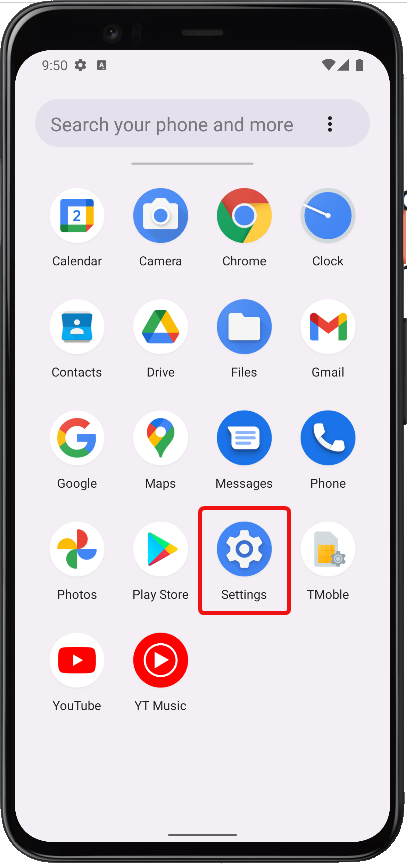This image appears to be a graphic mock-up of an Android phone screen. At first glance, it seems to capture a typical smartphone interface but closer inspection reveals it to be an illustration rather than a photograph of an actual device. 

At the top of the screen, the status bar displays essential information: the time, which reads '9:50,' followed by icons for settings, the signal strength, Wi-Fi connectivity, network status, and battery level. The color scheme of the interface is predominantly light grey, with subtle variations for elements like the search bar, which is presented in a slightly darker grey and contains the placeholder text "Search your phone and more," accompanied by three vertical dots. 

Below this, a horizontal bar hosts an array of app icons, systematically arranged. The apps included are: Calendar, Camera, Chrome, Clock, Contacts, Drive, Files, Gmail, Google, Maps, Messages, Phone, Photos, Play Store, Settings, T-Mobile (erroneously written as 'T-M-O-B-L-E'), YouTube, and YouTube Music.

A distinctive red box is drawn around the 'Settings' icon, likely to draw attention for instructional purposes, suggesting that the viewer click on 'Settings' for a specific task, possibly as part of a tutorial or guide on managing phone settings. The design and layout, combined with the iconography, strongly indicate that this is an Android phone interface mock-up.